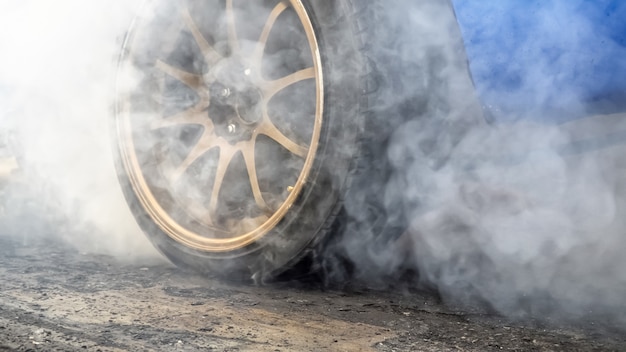The photograph vividly captures a car in the midst of performing a burnout on a rough, debris-strewn pavement, with the ground appearing either wooden or cement-like. Dominating the scene is a tire with an ornate gold, multi-spoke rim, set against the backdrop of the car's blue fender and black trim. Smoke billows dramatically around the tire, emphasizing the intense action and friction against the ground. The blue car occupies the upper right quadrant of the image, while the tire, central to the visual narrative, spreads from the middle to the lower left, giving a dynamic sense of motion and energy. The vividness of the image almost allows one to smell the burning rubber.